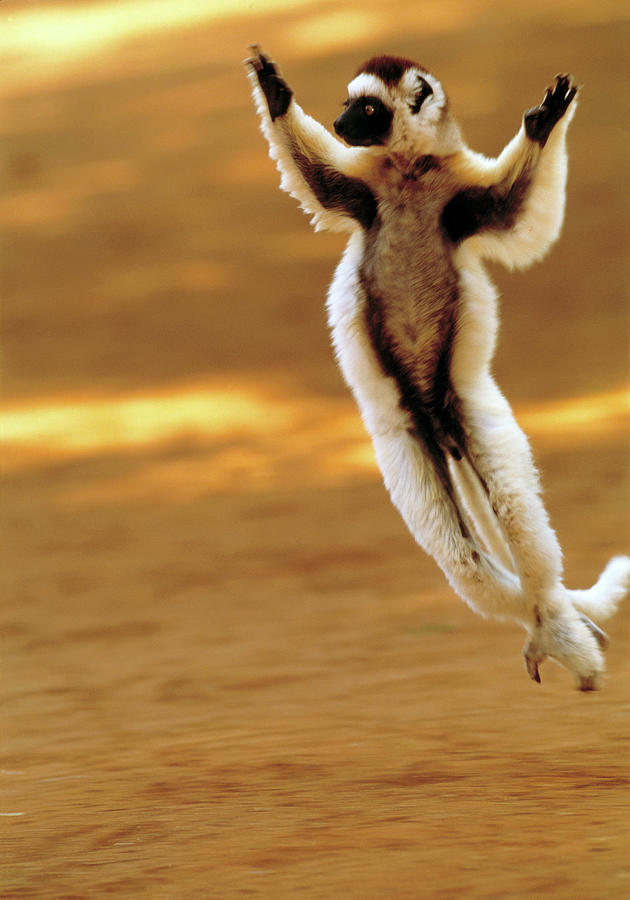The image captures a dynamic scene of a lemur in mid-air, either flying or leaping, set against an all-tan background that suggests sand, possibly hinting at a sunset or sunrise. The lemur, resembling Zoboomafoo, appears primarily white with a black face, black hands, and a white tail. It has a tan belly adorned with some maroonish-brown fur, providing a colorful contrast amidst golden, brown, and beige hues. The lemur's body is oriented in a three-quarter profile with its arms outstretched, fingers splayed, and bottom feet pointing downward. The close-up shot focuses on the lemur's expressive face, capturing the essence of its motion and the light from the sun illuminates the tranquil but vivid outdoor scene.